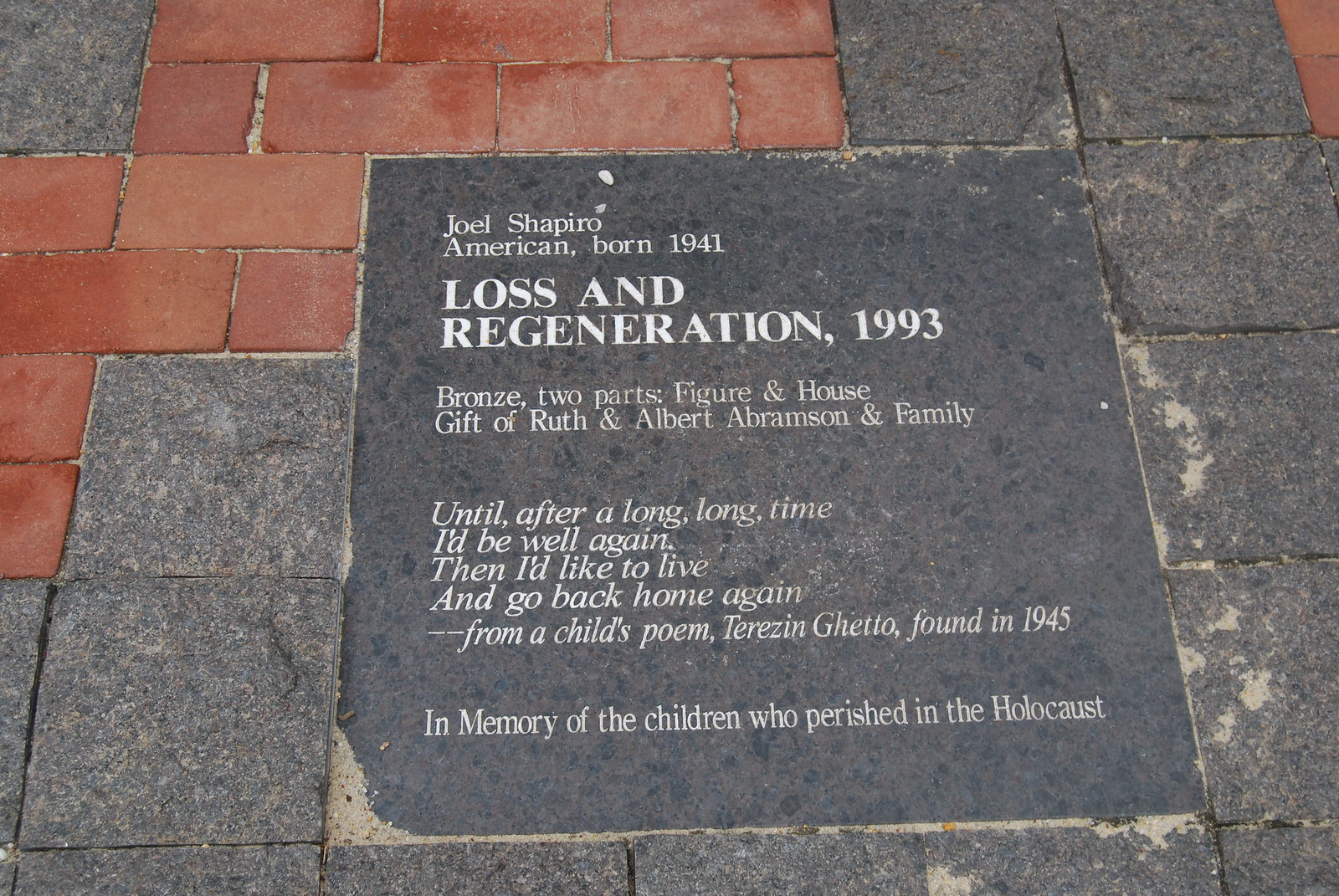This photograph captures a memorial plaque embedded in a brick and concrete walkway, featuring a mix of red and dark gray bricks. The plaque honors Joel Shapiro, an American artist born in 1941, and his 1993 bronze artwork titled "Loss and Regeneration," which consists of two parts: a figure and a house. This work was gifted by Ruth and Albert Abramson and their family. The plaque also includes a poignant quote from a child's poem, found in the Terezín Ghetto in 1945: "Until after a long, long time, I'd be well again, then I'd like to live and go back home," dedicated to the memory of the children who perished in the Holocaust.